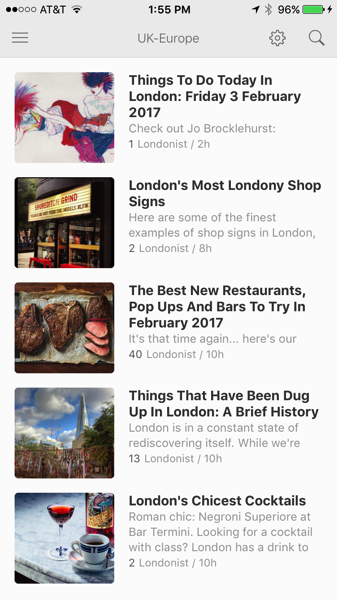This is a detailed screenshot of a mobile application interface. At the top of the screen, the status bar indicates the network provider as AT&T, with a Wi-Fi signal strength showing two out of five circles filled in black. The current time is displayed as 1:55 PM, and on the right side, there is a battery icon showing 96% with a green indication that it is charging. Additional icons for location and Bluetooth are also present.

Below the status bar, the app header shows "UK-Europe" with a settings icon and a search icon on the right, and a menu icon on the left. 

The main content showcases a series of stories accompanied by images:
1. The first article titled "Things to Do Today in London, Friday 3 February 2017" features a cartoon image.
2. The second article, "London's Most Londony Shop Signs," discusses some of the finest examples of shop signs in London, illustrated by a picture of a shop storefront.
3. The third article, "The Best New Restaurants, Pop-ups, and Bars to Try in February 2017," is accompanied by a photo of a steak.
4. The fourth article, "Things That Have Been Dug Up in London: A Brief History," includes a photograph of a building against the sky.
5. The final article featured is "London's Chicest Cocktails," with an image of a coffee and a cocktail side by side.